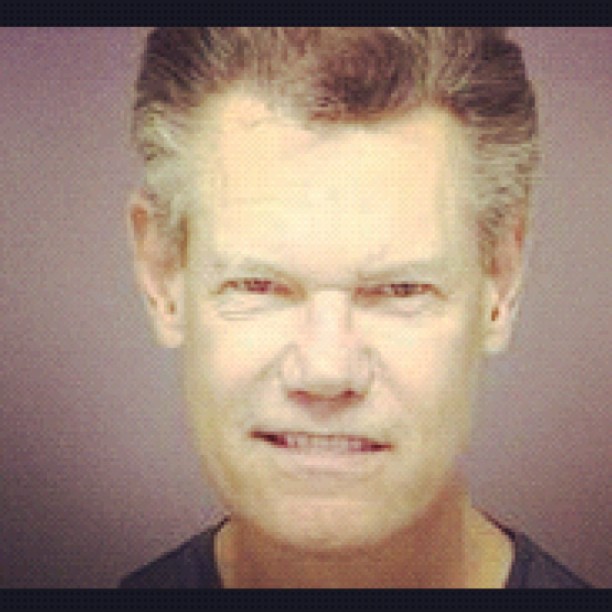This image is a square format color photograph featuring a close-up of a man resembling Randy Travis, a famous singer. The photograph is old and of poor quality, with a grainy texture and muted colors. The man, likely in his late 50s, is an older Caucasian male with dark brown hair speckled with gray, cut very short. He is looking directly at the camera with a facial expression that combines a slight smile and a possible grimace or scowl, revealing the top row of his teeth. His eyes are somewhat closed, with noticeable wrinkles underneath. The image is cropped tightly, cutting off the top of his head and extending just below his neck, showing the tops of his shoulders. He is wearing a dark blue or black t-shirt. The background is an indistinct, blurry gray, possibly with a rose color gradient, and there are black borders at the top and bottom. The entire photograph has a lot of glare, particularly on his forehead and cheekbones.